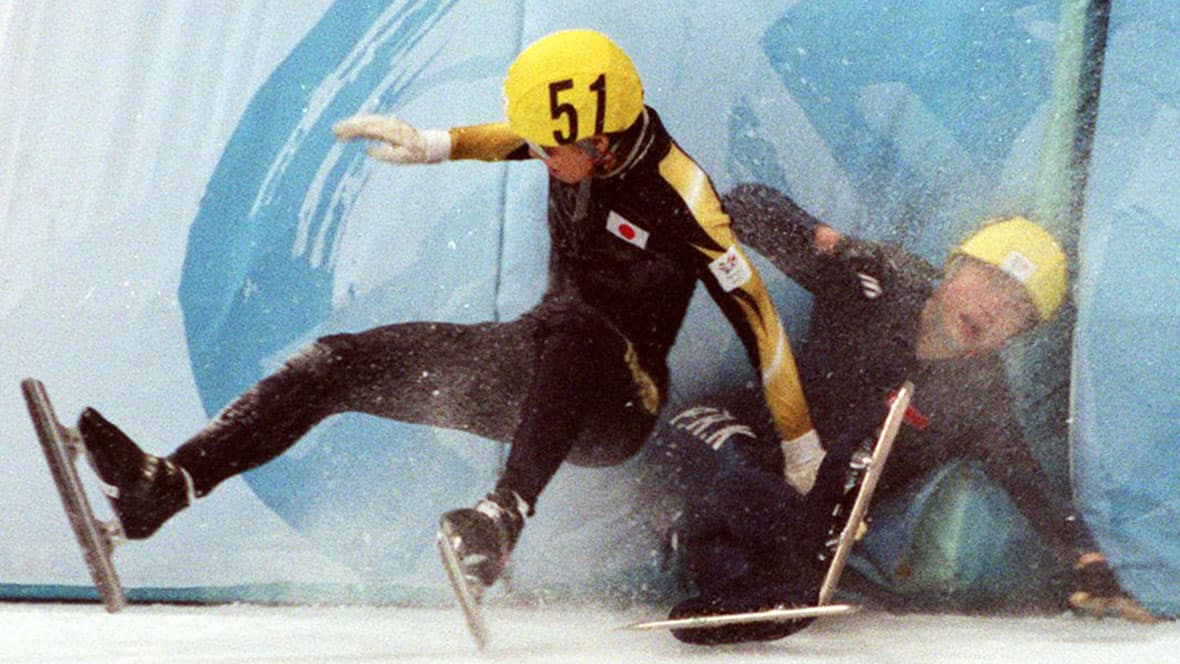This photograph captures a dramatic moment at a sporting event, featuring two speed skaters mid-crash on an icy rink. Both athletes are adorned in black speed skating leotards with long yellow sleeves and matching yellow helmets. One skater, sporting the number 51 on his helmet, bears the flag of Japan on his uniform, highlighting his nationality. This skater is already on the ground, legs splayed out in front of him, with one hand bracing against the ice. The other skater, also wearing a yellow helmet and white gloves, is caught in the act of falling, with his feet slipping out from under him, yet his hand has not yet reached the icy surface. Their silver skate blades gleam against the cold, blue ice, adding to the sense of motion and impending impact. The scene is set against a light blue wall, emphasizing the skaters' struggle and the intensity of the moment.